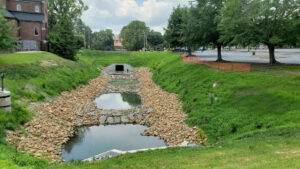This horizontally aligned rectangular image depicts an outdoor scene centered around a small drainage ditch or creek. The ditch, lined with rocks predominantly toward its edges, contains a couple of large puddles, giving the appearance of having been partially drained. The rocky terrain leads to a visible ground drain or culvert at the center, suggested to go under a pathway or street.

Flanking the ditch on both sides are slight inclines covered in lush green grass. To the left of the image, in the upper left corner, there's a two-story brown or reddish-brick building with more of it off-frame. On the upper right side, there's a greyish parking lot, devoid of cars, and surrounded by trees. In the background, amidst the trees, another building can be faintly seen. Completing the scene, the sky at the top of the image features large, puffy gray and white clouds, adding depth and ambiance to the serene setting.